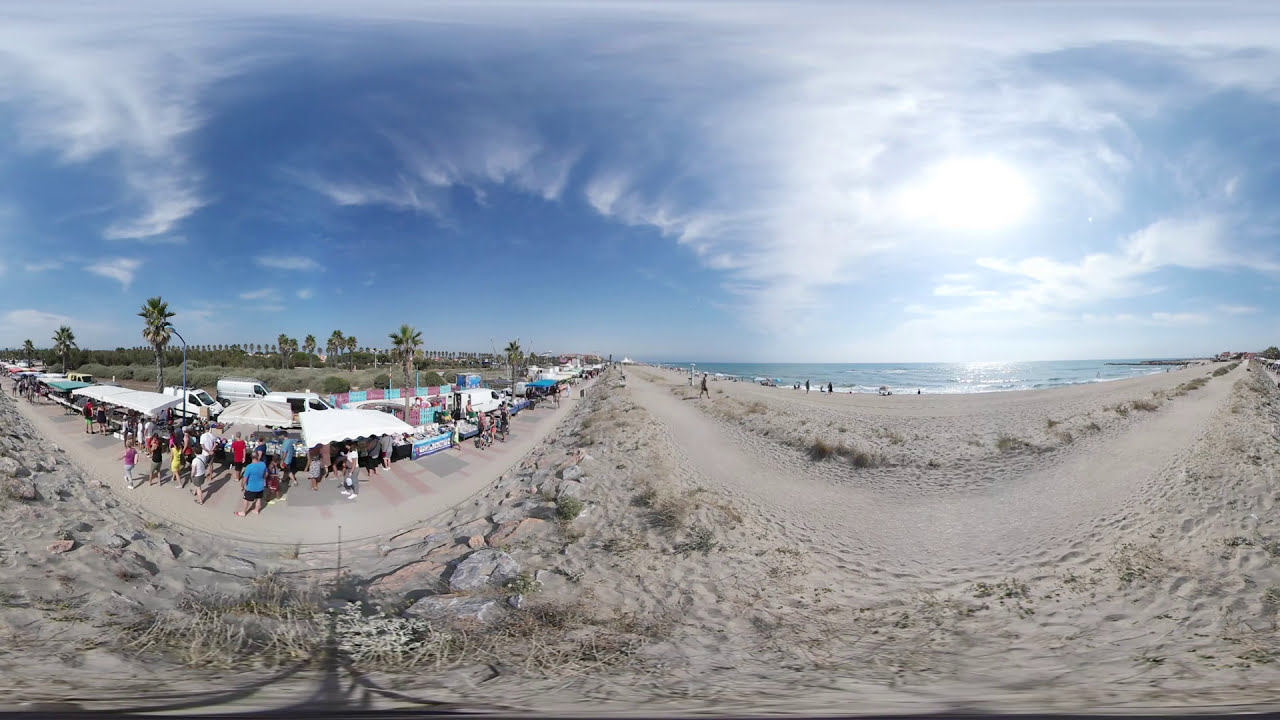This image captures an outdoor beach scene, likely taken through a double fisheye lens, which creates circular distortions in the frame. The foreground is dominated by a sandy beach interspersed with beachside vegetation such as scrub brush. To the left, there is a bustling area filled with numerous tents and pavilions, suggesting an event like a farmer's market or a similar gathering. People clad in colorful vacation attire can be seen milling around the tents. The background features palm trees and perhaps coconut trees, indicating a tropical or subtropical location, potentially in California or Florida. The right side of the image displays the ocean with deep blue waters, and mid-afternoon skies feature streaky, white clouds. Some people are also visible near the water, enjoying the beach. Overall, this lively and vivid scene is framed by a blue, hazy sky that seamlessly merges with the landscape and the lively activity below.